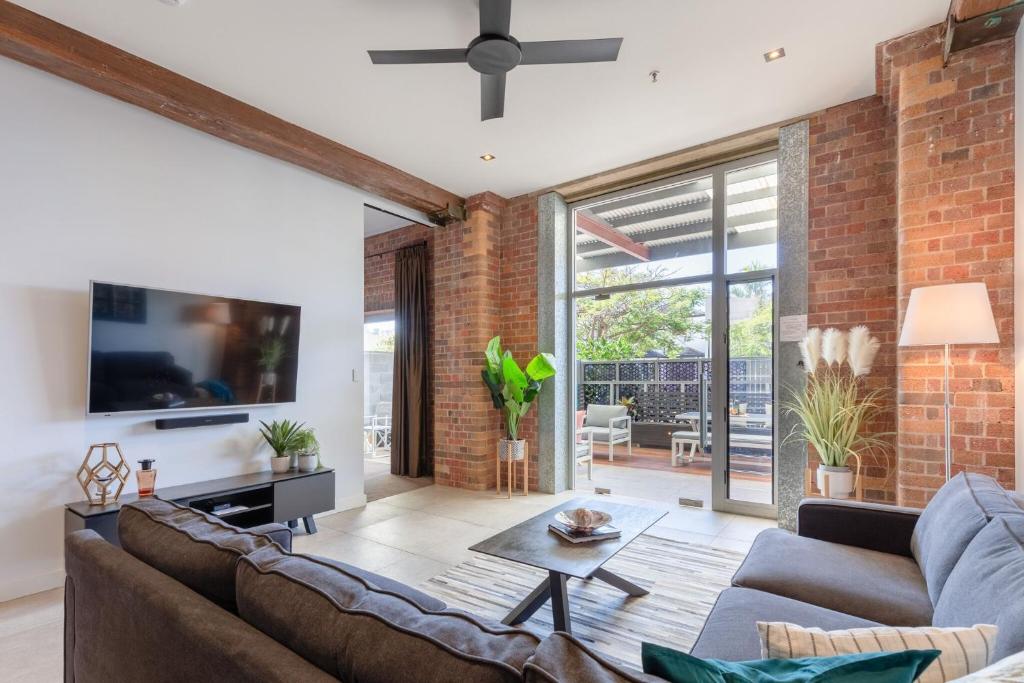The photograph of the room showcases a stylish and modern interior, likely used for real estate listings or promotional purposes. The room features a large living area with gray fabric sofas including a sectional L-shaped couch adorned with blue and white throw pillows. Centrally located is a sleek, modern coffee table on a light-striped rug, with a book placed on it. 

The wall to the left is white and houses a large flat screen TV, underneath which sits a black, low-lying table decorated with potted plants. Above the TV, a brown wooden beam connects the wall to the gray-painted ceiling, which is also complemented by a black ceiling fan. The adjacent wall to the right is constructed with vivid orange and red bricks, adding a touch of rustic charm.

A prominent feature of the room is the large sliding door leading out to a patio furnished with outdoor furniture. The patio is framed by windows and overlooks a scenic view of trees. Flanking the sliding door are two potted plants in white pots supported by wooden legs, each containing green foliage accented with five white stems. Additionally, the space includes corner lighting with a white lamp and minimalistic decorations, maintaining a clean, contemporary, and inviting aesthetic.